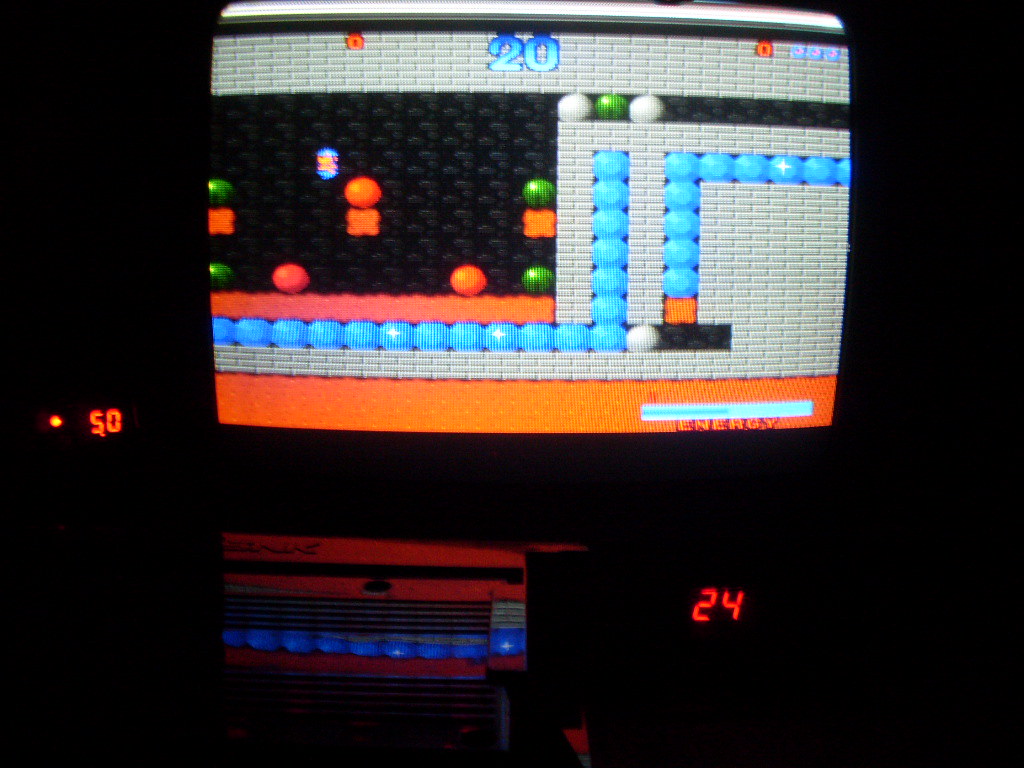The image features a screen with a black background, showcasing an illuminated rectangle at its center, which appears to be displaying a game. The game screen resembles a classic Mario level, characterized by traditional gray blocks and red lava beneath them. A green energy bar with red text is visible at the bottom right corner of the game interface. Below the screen is a system that seems to be powering the display, likely a game console. To the right, there are numbers displayed in an analog format, specifically the number "24" in red. Additional red numbers are located to the upper left of the screen. The game display shows a small character navigating through an environment filled with circles and squares.